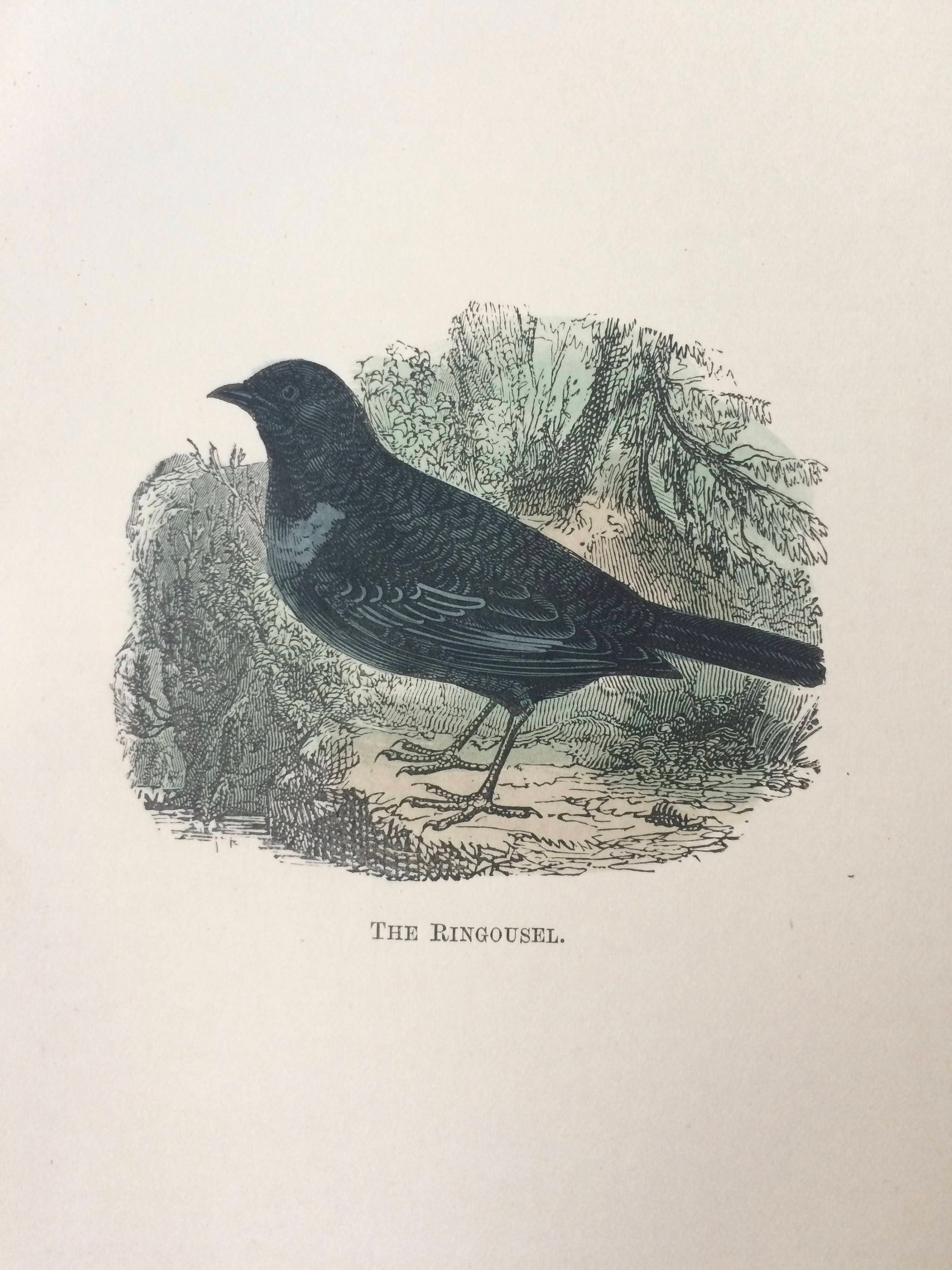This illustration depicts a detailed drawing of a bird labeled as "Ring Ouzel." The bird, primarily black with a dark gray underbelly and some dark blue elements on its feathers, is standing upright on its two legs. Its short beak and distinct feather patterns are reminiscent of illustrations in old nature books or scientific journals. The bird is shown facing left, with its tail pointing to the right, amidst a backdrop of green vegetation and leaves, suggesting a forested environment. The background is set on a cream-colored, paper-textured enclosure that is irregularly shaped and focuses on a localized area of the bird's habitat. The vintage color palette and articulate details highlight the bird's specific physical characteristics, making the illustration appear both classic and meticulously crafted.